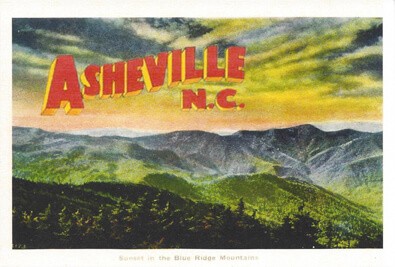This vintage postcard, possibly from the 1950s or 60s, features a horizontally oriented, hand-painted mountain scene. The postcard, bordered by slightly yellowed off-white edges, showcases a serene landscape with gray mountains stretching across the center. In the foreground, rolling green hills dotted with pine trees add a vibrant contrast. Above, the sky displays a mesmerizing blend of reddish, yellow, and blue hues, reminiscent of a sunset, with puffy cirrus clouds adding texture. In the top left corner, the words "Asheville, N.C." are prominently displayed in large red block letters with a yellow background, emphasizing its nostalgic charm. The overall style of the artwork is soft, using pastel and watercolor techniques to evoke a sense of tranquility and timeless beauty.